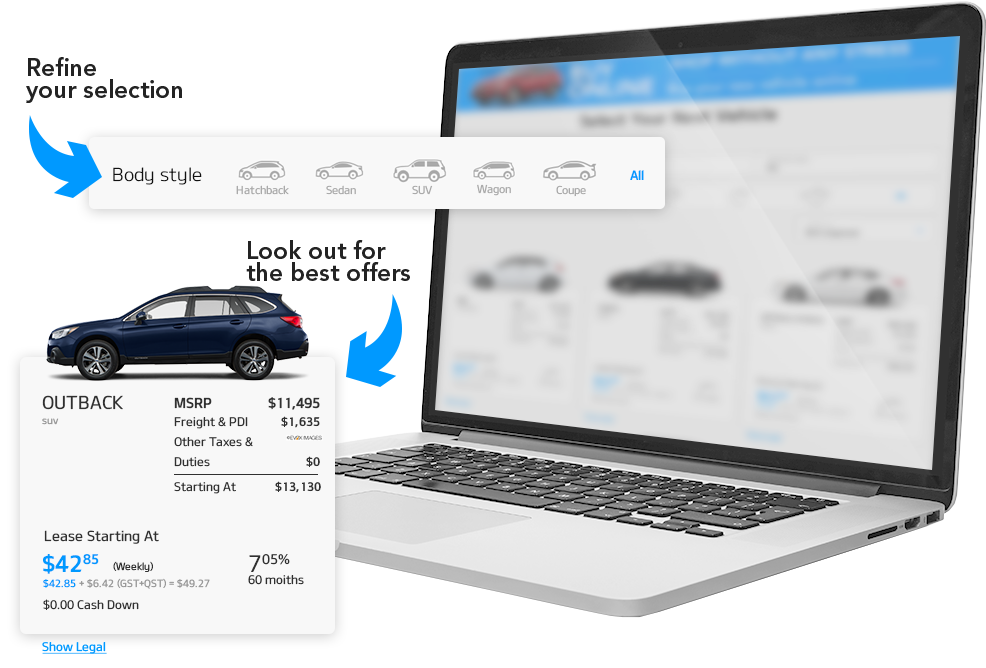This detailed screenshot captures a simplistic yet functional layout of a car purchase or leasing website, likely viewed on a PC or tablet. The background is plain white, enhancing the clarity and visibility of the elements. 

On the left side of the screen, there's an open laptop, oriented towards the left, showcasing what appears to be a blurry car search interface. Dominating the top left corner, the heading "Refine Your Selection" is printed in black. Below this heading, a prominent blue arrow directs attention downward to a section that helps users select a car body style. This section includes labeled diagrams of various car types, such as Hatchback, Sedan, SUV, Wagon, and Coupe.

Further down, black text instructs, "Look out for the best offers," complemented by another blue arrow, indicating a featured area. This highlighted section contains an image of a black SUV, specifically a CRV model, marked with the label "Outback," SUV. Below the image, detailed information about the car is provided in dark blue text set against the white background. All textual and graphical elements are neatly arranged within a square feature situated under the car image, maintaining a clean and organized appearance that complements the overall website design.